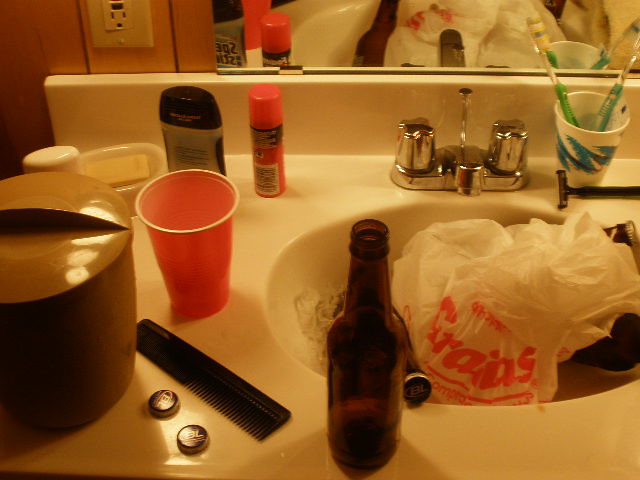The image depicts a cluttered bathroom sink adorned with a variety of colorful items. On the sink's surface, a white cup with blue decorations holds two green and white toothbrushes. Surrounding the cup is a black razor placed directly in front of it. A white plastic shopping bag rests inside the sink basin.

Nearby, there are two bottles of alcoholic beverages; one bottle is placed inside the sink while the other stands right outside the sink bowl. To the left of the external bottle, there is a black hair comb positioned adjacent to two bottle caps, presumably from the alcoholic drinks.

Additionally, a red drinking cup sits above the hair comb, while to its right, an orange personal care spray—potentially shaving cream or perfume—stands beside a black and gray container. Completing the ensemble, a bar of soap is placed next to the personal care items, and a brown ceramic container is situated near the black comb.